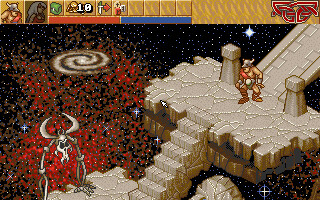The image is a rectangular screenshot depicting a dynamic scene from a stylized, fantastical video game. The top portion of the screen features a series of small, golden boxes, each adorned with various icons and one marked with the number "10," suggesting clickable in-game options or inventory items.

Beneath these golden boxes, a segmented band of vivid orange transitions into a blue section under four of the unadorned gold boxes. In the upper right corner, a striking red, twisted emblem stands out, hinting at a significant game element or status indicator.

The mid-ground of the scene showcases a detailed environment with two distinct creatures positioned in different areas. One creature, depicted upright, ascends a set of stairs that lead to a grayish-tan platform. Adjacent to this platform, there's a ramp leading upward. Above and beyond this setting, a mesmerizing visual effect resembling a swirling vortex graces the starry backdrop, painted black with sporadic patches of red.

Additionally, a skeletal figure with prominent horns occupies a lower platform, integrated seamlessly into this otherworldly, visually rich gaming universe. Stars scattered throughout the background add depth and emphasize the fantastical theme of the game.